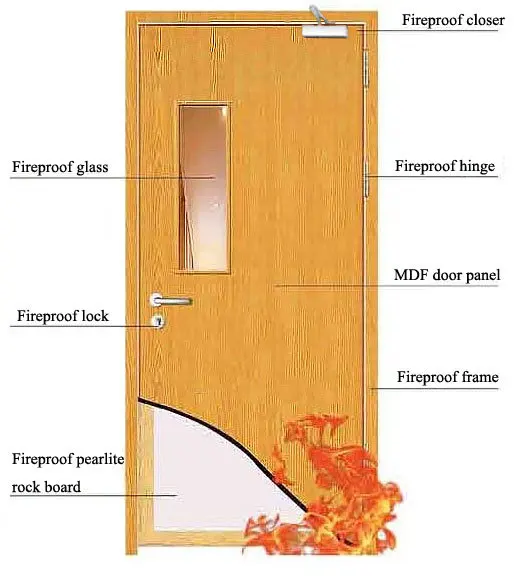The image depicts a brown wooden door with distinct vertical grain patterns. It has a narrow, vertical rectangular window cutout on the left side labeled "fireproof glass." Directly below the window is a silver pole handle with a lock beneath it, indicated as a "fireproof lock." The door is set against a completely white background, with various descriptive labels pointing to its key features. At the top of the door is a silver object marked as "fireproof closer," connected to by an arrow. The middle of the door is denoted as an "MDF door panel," and the frame surrounding it is tagged as "fireproof frame." The hinges on the right side are specified as "fireproof hinge." The lower left corner of the door panel reveals an inner white or light gray layer called "fireproof pearlite rock board," which is partially exposed. In front of the door, in the bottom right corner of the image, flames are depicted, symbolizing the door's fire-resistant properties.